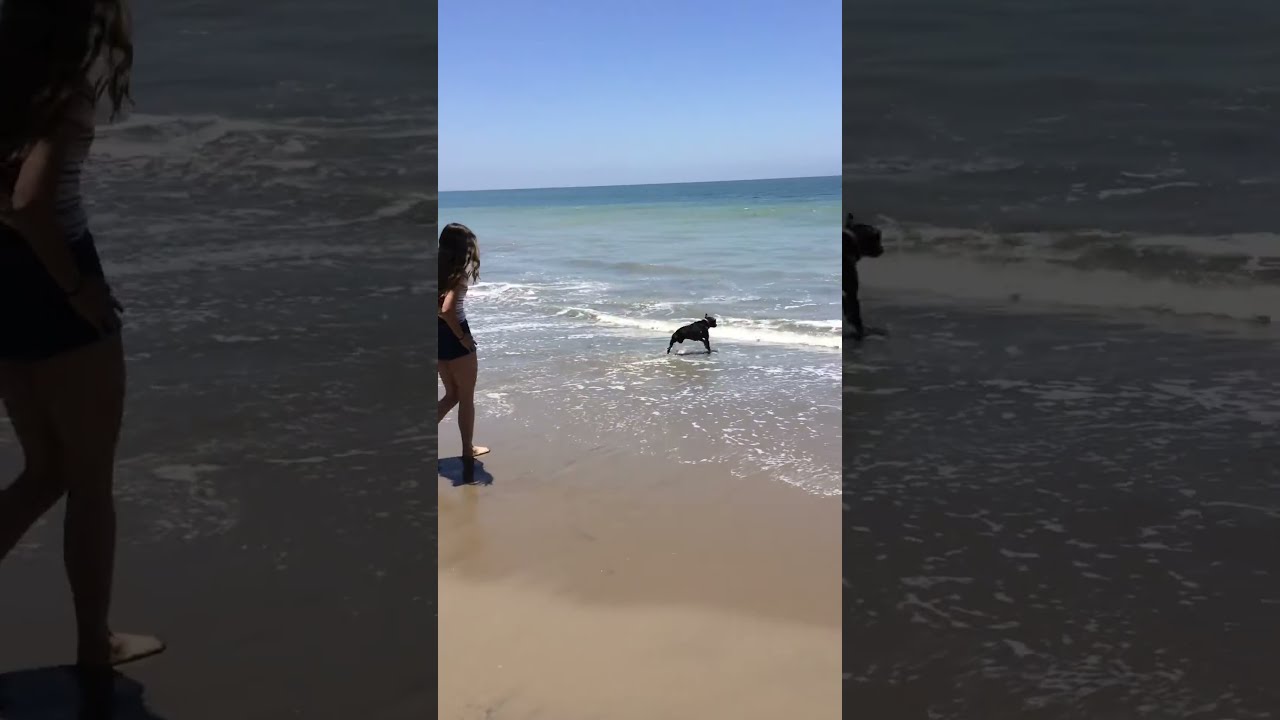In this beach scene, a young, tanned, athletic girl with long dark hair walks along the grayish-brown sand at the ocean's edge. She is on the left side of the image, dressed in dark shorts and a light-colored top. The gentle surf, about 10 inches high, laps at her feet, and the water transitions from a foamy white at the shore to a blue-green hue before deepening into a rich blue further out. A small, black dog plays exuberantly in the shallow water, darting back and forth among the waves, one of its ears flapping up. The sky above is a light blue, complementing the serene seascape. The horizon shows a ridge, suggesting the beach could be part of an inlet. The overall image has a wide border created with enlarged, grayed-out elements from the main scene to frame the picture.